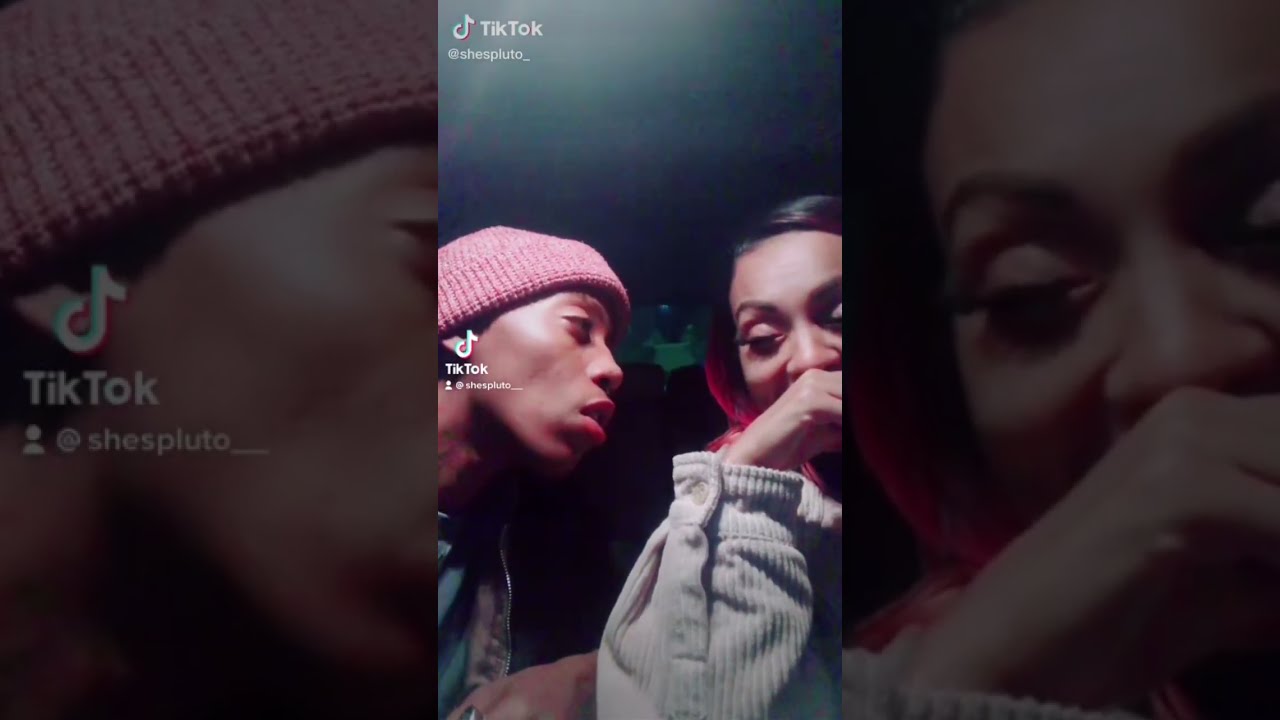This image is a detailed screenshot from a TikTok video by user @shespluto_ with the TikTok watermark appearing in the top left corner, as well as the username and logo displayed mid-way down the left side. The image features a black man and woman who appear to be in a car. The man, positioned on the left-hand side, is wearing a light red beanie and a t-shirt under an overshirt. He is facing the woman with an expression that suggests he has just spoken, as his mouth is slightly open and he looks serious. The woman, on the right-hand side, has dark hair with red streaks near the bottom and is wearing a white corduroy jacket. She appears to be laughing, covering her mouth with one hand while her eyes are closed. The background of the image suggests they are in a car, indicated by a baby car seat visible at the bottom and a grayish color at the top. The borders of the image have been blurred, taking up a significant portion of the frame.